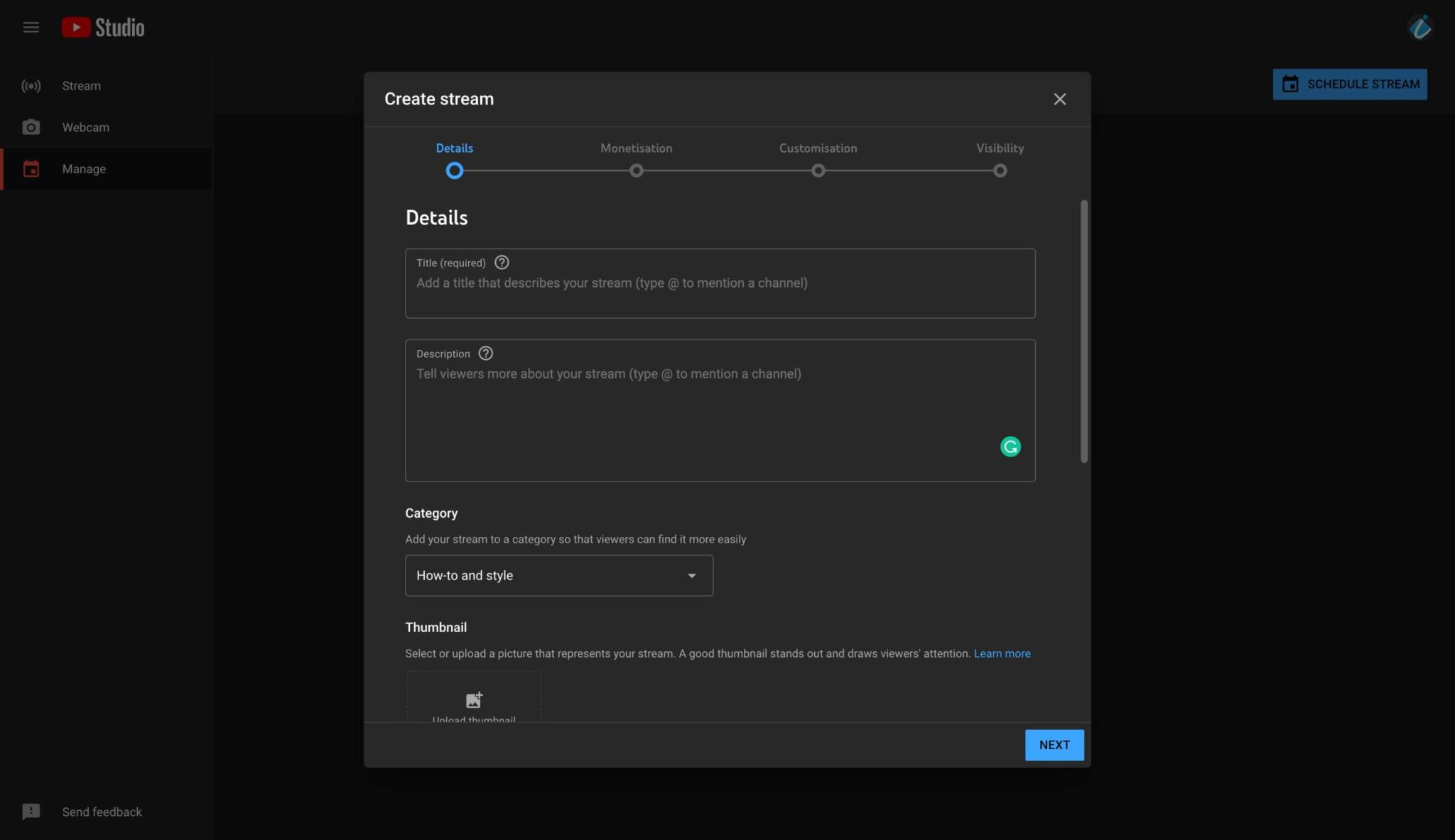The image depicts a user interface of a live streaming setup. In the top right corner is a black section featuring a prominent red box with a white arrow pointing to the right, beside a large white text spelling out "STUDIO." Below this, a vertical menu on the left lists options like "Stream," "Webcam," and "Manage," each accompanied by icons in adjacent columns. 

Dominating the center of the screen is a sizable gray box. At the upper left corner of this box, the white text reads "Create Stream," with the subsequent lines displaying the labels "Details" and a blue button and blue text also labeled "Details." Further down, the center is segmented by white text headings such as "Monetization," "Customization," and "Visibility."

Under the "Details" section heading on the left, there is an input box meant for stream information, followed by another labeled "Description," which prompts users to "Tell viewers more about your stream." Below this, a "Category" section instructs users to add their stream to a category to facilitate easier discovery by viewers. Near the bottom, under the "Thumbnail" section, advice is given to "Select or upload a picture that represents your stream," emphasizing that a good thumbnail captures viewer attention; additionally, a link labeled "Learn more" is provided in blue text. On the bottom right of the gray box, a blue button with black text is labeled "Next."

Overall, the visual presentation effectively outlines the steps and components involved in setting up a live stream, providing clear guidance and options for user customization.